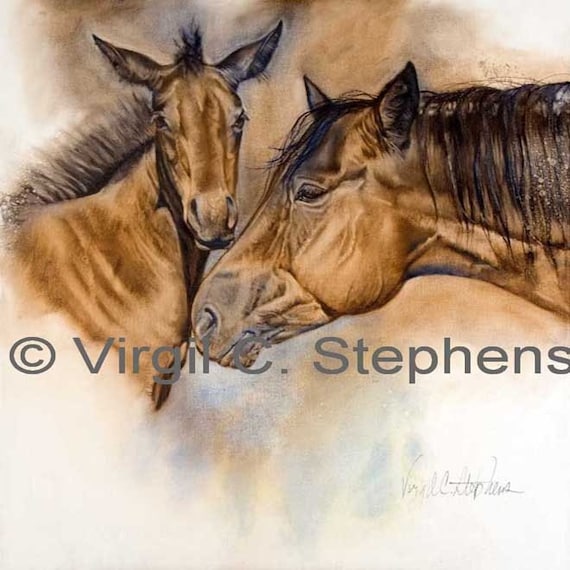This image is a watercolor painting by Virgil C. Stevens, who has both signed and copyrighted the piece, his credentials visible in the middle and the bottom right of the painting. The artwork features two brown horses with black manes. The larger horse stands on the right, presenting a muscular, veiny face with a long snout. Its mane is flowing down towards its eye, giving it a mature, weathered appearance. The smaller horse to the left appears more youthful, with a shorter face and mane standing upright. This horse is looking directly forward, while the larger one gazes off to the left. The background consists of a smudged mixture of brown, black, white, and hints of darkish blue, which contrasts with the hyper-realistic details of the horses and enhances the overall aesthetic. The lack of bridles suggests a sense of natural freedom in these majestic animals.